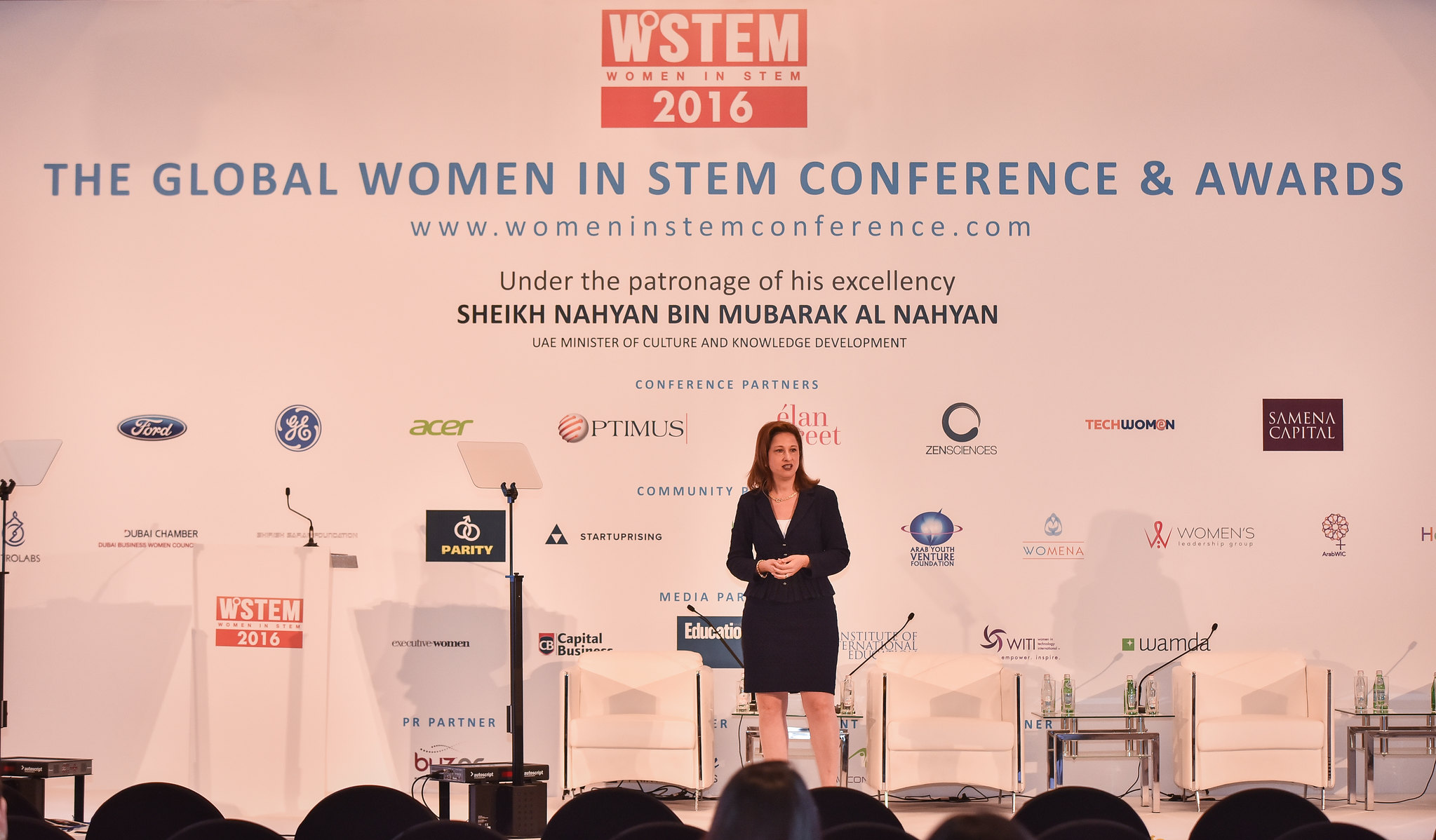The image captures an indoor conference setting with a woman on stage, addressing an audience whose heads are visible at the bottom of the frame. The woman, dressed in a black suit jacket over a white shirt and a black skirt, stands with her hands crossed in front of her. She has shoulder-length brown hair and is looking to the right. Behind her is a white banner with several layers of text. At the top, in a red section, it states "WSTEM Women in STEM 2016," followed by blue text announcing "The Global Women in STEM Conference and Awards." Below, it displays the website "www.womeninstemconference.com." Further down, in black text, it mentions the patronage of "His Excellency Sheikh Nahyan bin Mubarak Al Nahyan, UAE Minister of Culture and Knowledge Development." At the bottom, there is a list of conference partners, including brands such as Ford and Acer. The stage features three cream-colored chairs and two tables, with a podium off to her left, completing the setting for this formal presentation.